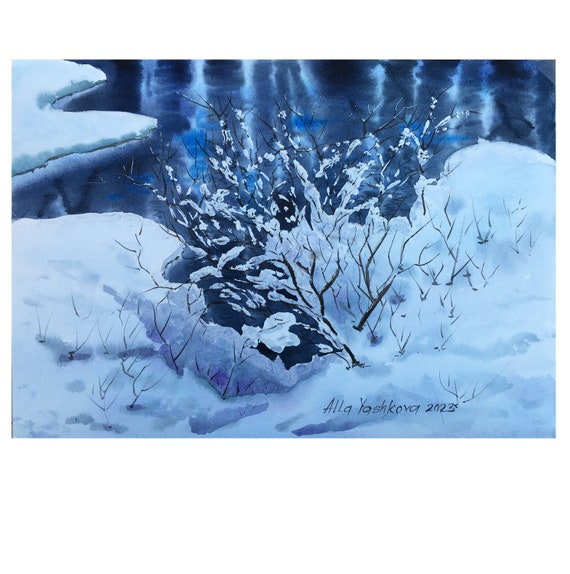This captivating digitally generated or animated image, signed "Ela Yashkova 2023" at the bottom right, showcases a serene, snow-covered landscape dominated by shades of blue. It features a small, almost dried-up tree or shrub without leaves, centrally positioned on a rocky, snow-capped terrain. The branches are dotted with clusters of snow. The backdrop presents a dramatic contrast with dark, glossy blue hues suggesting a water feature, possibly a lake or a waterfall mingling with the snowy surroundings. The sky is depicted as a deep, night black, enhancing the stark beauty of winter. The artistic style combines elements of realism with a glossy, vibrant touch, making the scene vivid and lifelike.